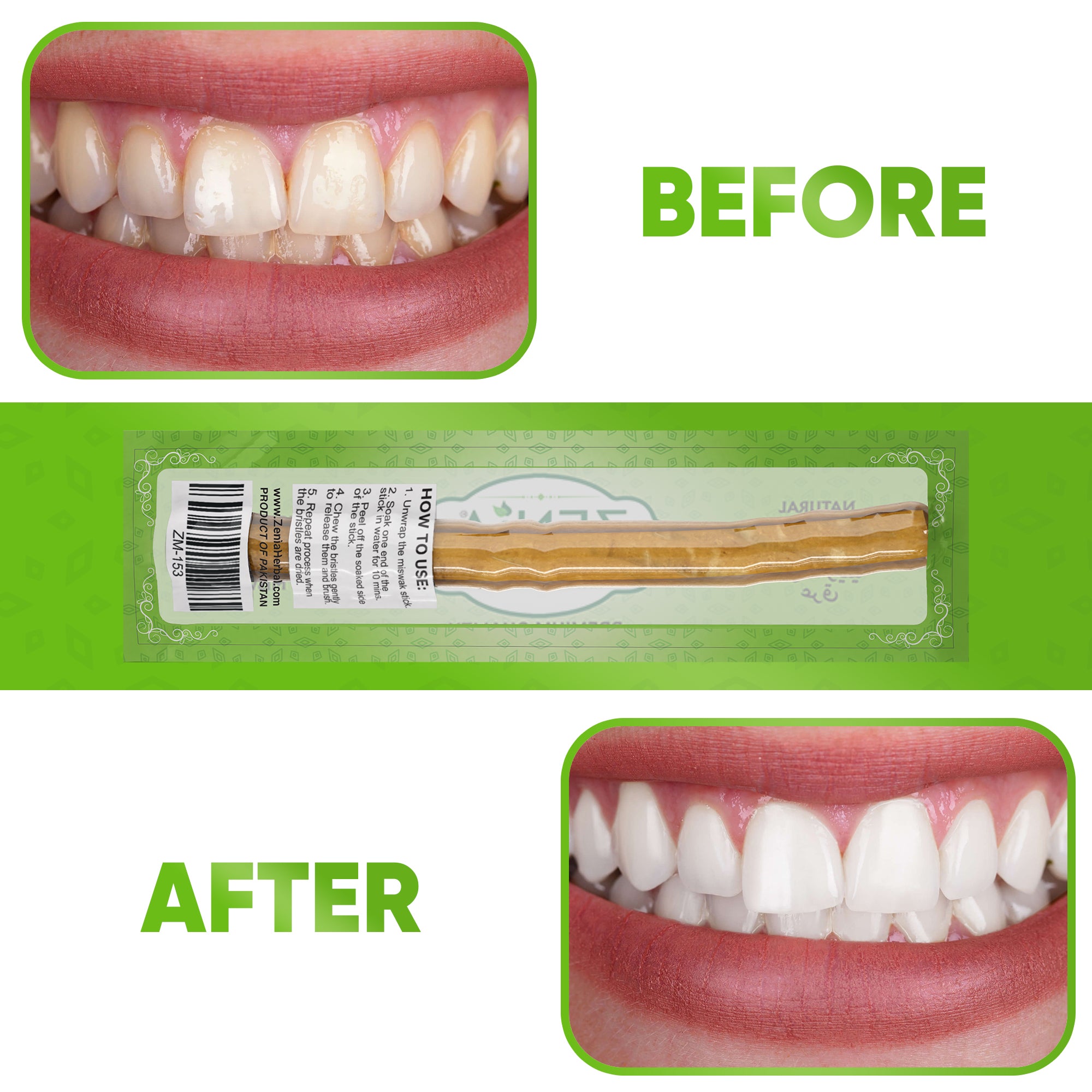This image shows a dental care product packaged in a green-bordered wrapper adorned with leafy designs. The focal point of the package includes a "before" and "after" image of teeth, with green lettering indicating "before" and "after." The "before" image depicts a slight smile featuring pink lips and gums, with teeth showing yellowing primarily along the edges near the gum lines. The "after" image reveals significantly whiter, healthier-looking teeth.

In the center of the package, a brown, stick-shaped dental device is visible, known as a mishwax stick. Instructions for use are printed below the device, explaining that the stick should be unwrapped, one end soaked in water for 10 minutes, then peeled to reveal a bristle side, which should be gently chewed to release the bristles for brushing. This product, identified as being made in Pakistan, is designed to clean and whiten teeth, with a clear visual demonstration of its effectiveness through the "before" and "after" photos.